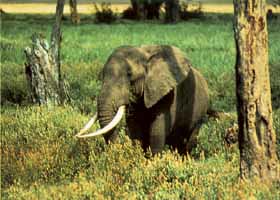In the picture, a prominent gray elephant with long, white tusks stands in a field. The elephant, positioned centrally, gazes into the distance. Surrounding the elephant is a mix of taller grasses and thicker, yellow-tinted brush partially obscuring its trunk. To the elephant's left is a tree stump, while to its right stands a light brown tree trunk providing a bit of shade, though the shading is light due to the sparse foliage. The background features a lush green field stretching into the distance, dotted with occasional tree trunks and rocky structures. This daytime scene captures sun rays illuminating various parts of the landscape, adding to the natural ambiance of the setting. No other elephants or significant objects are visible, keeping the focus on the solitary, majestic creature in its serene environment.